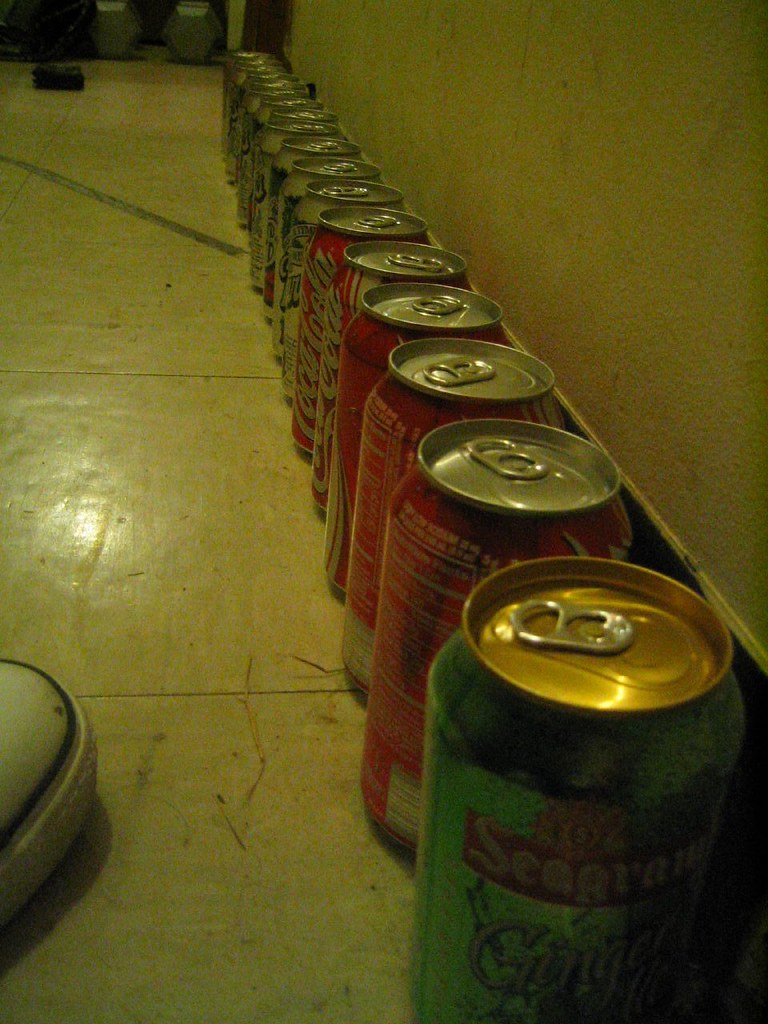In this dimly lit room with a dirty, yellowish-white tile floor, an array of unopened soda cans lines up against the wall, diminishing in size into the distance. The sequence starts with a green Seagram's ginger ale can closest to the camera on the right. Following it are several Coke and Barq's root beer cans, and additional unidentifiable cans continue off the frame. The cans angle slightly to the left as they recede. The wall behind them is similarly yellowish-white, matching the floor's grime. In the bottom left corner of the image, part of a Converse-style low-top shoe is visible, identifiable by its black sole and white toe. The scene also includes a piece of tape on the floor and a glimpse of two dumbbells and a door in the background.